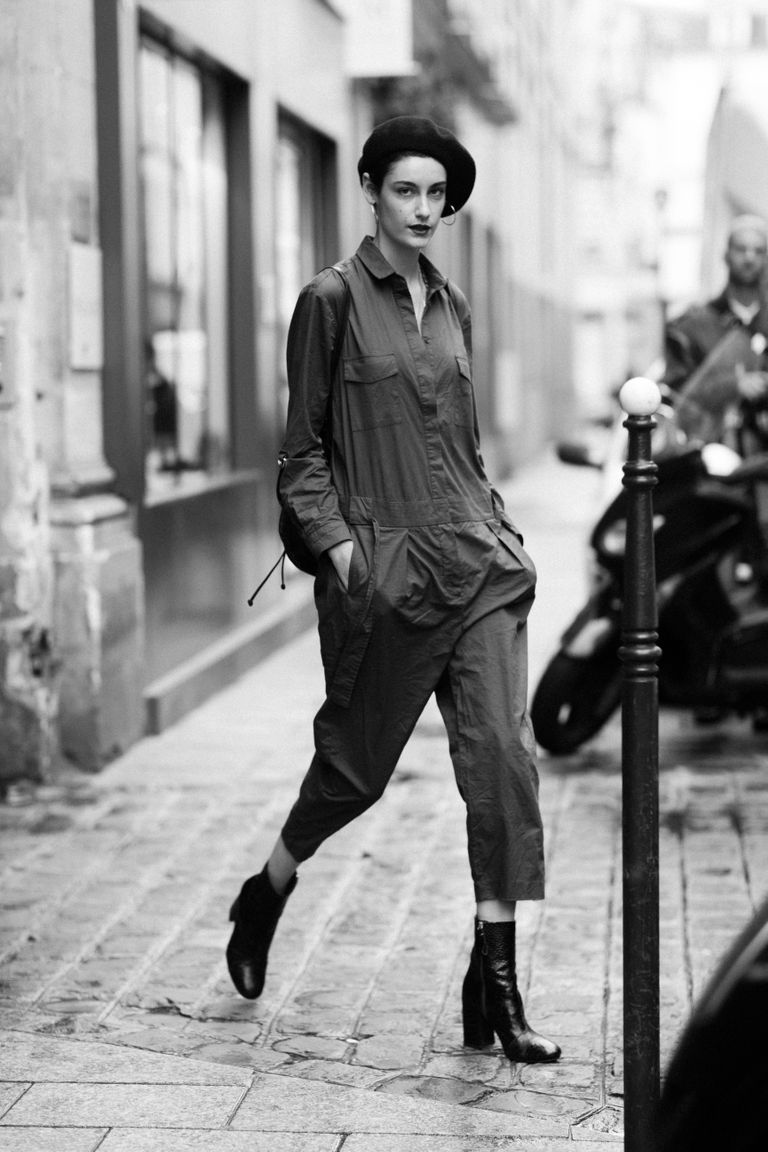This black-and-white photo captures a striking scene of a woman walking left to right on a stone sidewalk in front of a storefront. She is donned in a dark-colored, slightly baggy jumpsuit that zips up the middle, featuring a collar and long sleeves. The jumpsuit's pant legs cut off mid-calf, exposing a sliver of skin above her black heeled boots. Her short hair is topped with a dark beret, and she accessorizes with hoop earrings. The woman is angled toward the camera, confidently striding forward.

In the background, a row of motorcycles lines the street, and a man is seen standing behind one of the motorcycles, though his figure is blurred due to the depth of field. The background also includes a stone building with two visible windows to the left and a black pole with a white ball on top situated at the forefront on the right. The overall composition radiates a vintage charm, underscored by the monochrome color scheme.